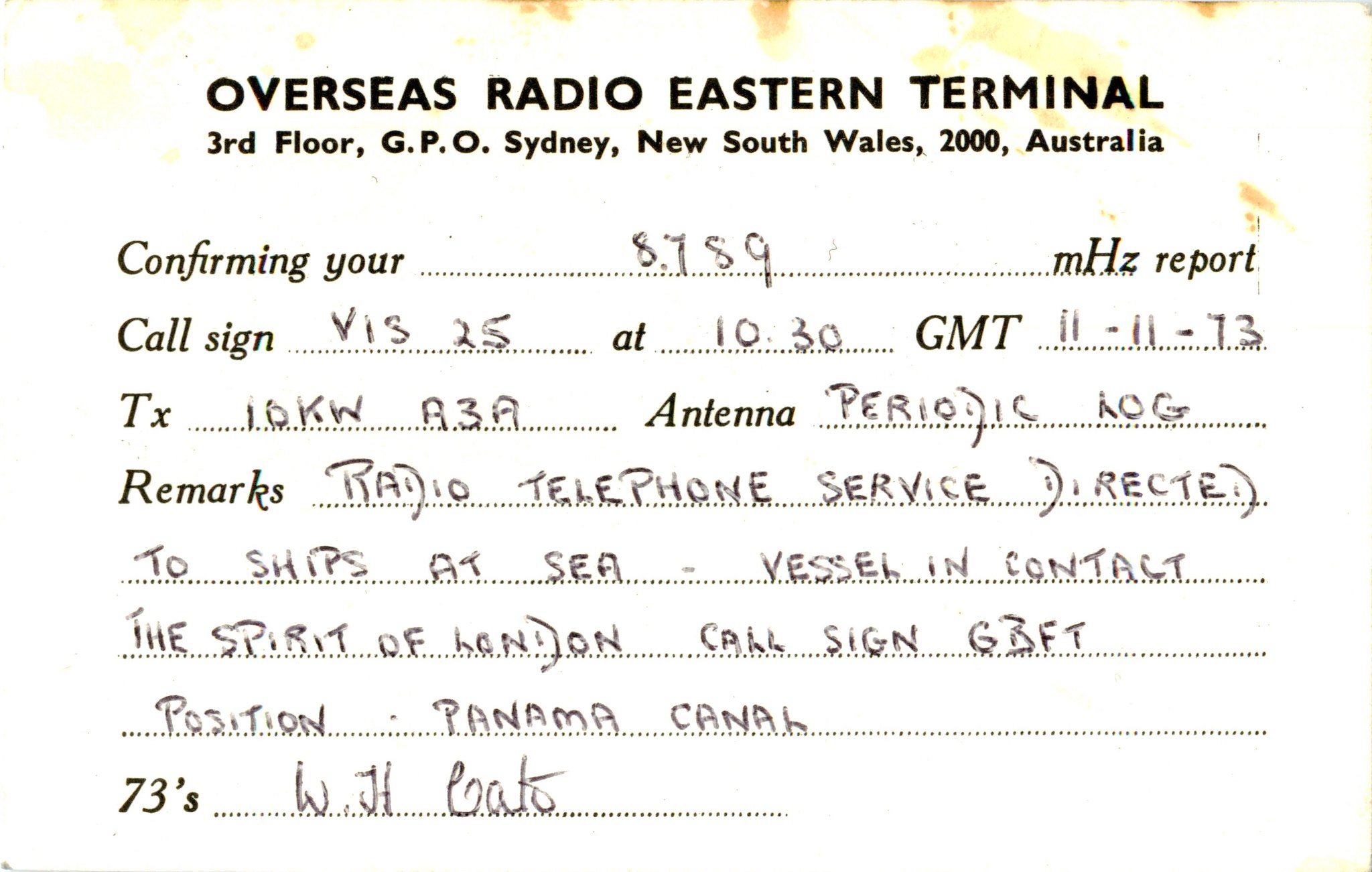This rectangular image, wider than it is tall, has a degraded white background marred with yellow and brown discolorations, indicating its age. Despite the faded outline, the clarity and structure of the content remain visible. The top of the image features bold black print that reads, "Overseas Radio Eastern's Terminal." Below that, also in bold black print, is the address, "Third Floor, GPO Sydney, New South Wales 2000, Australia."

The document includes several pre-printed sections with dotted underlines meant for filling in information. In these sections, handwritten text in black ink provides details as follows:

- Pre-printed: "Confirming your," with handwritten fill-in: "8789." 
- Pre-printed: "M Hertz report call sign," with handwritten fill-in: "V 1 3 2 5."
- Pre-printed: "at," with handwritten fill-in: "1030."
- Pre-printed: "GMT," with handwritten fill-in: "11-11-73."
- Pre-printed: "TX," with handwritten fill-in: "10 KW A 3 A."
- Pre-printed: "Antenna," with handwritten fill-in: "Periodic AOG."

In the "Remarks" section, handwritten information in black ink states: "Radio Telephone Service directed to ships at sea. Vessel in contact: The Spirit of London, call sign GBFT, position Panama Canal." The pre-printed "73's" is followed by a handwritten signature that ambiguously reads, possibly, "WH CATS" or "WH COATS."

The image seems to capture a historical communication document, likely used for maritime radio transmissions, showcasing both the pre-printed format and personalized handwritten details that together relay a precise log entry from the past.